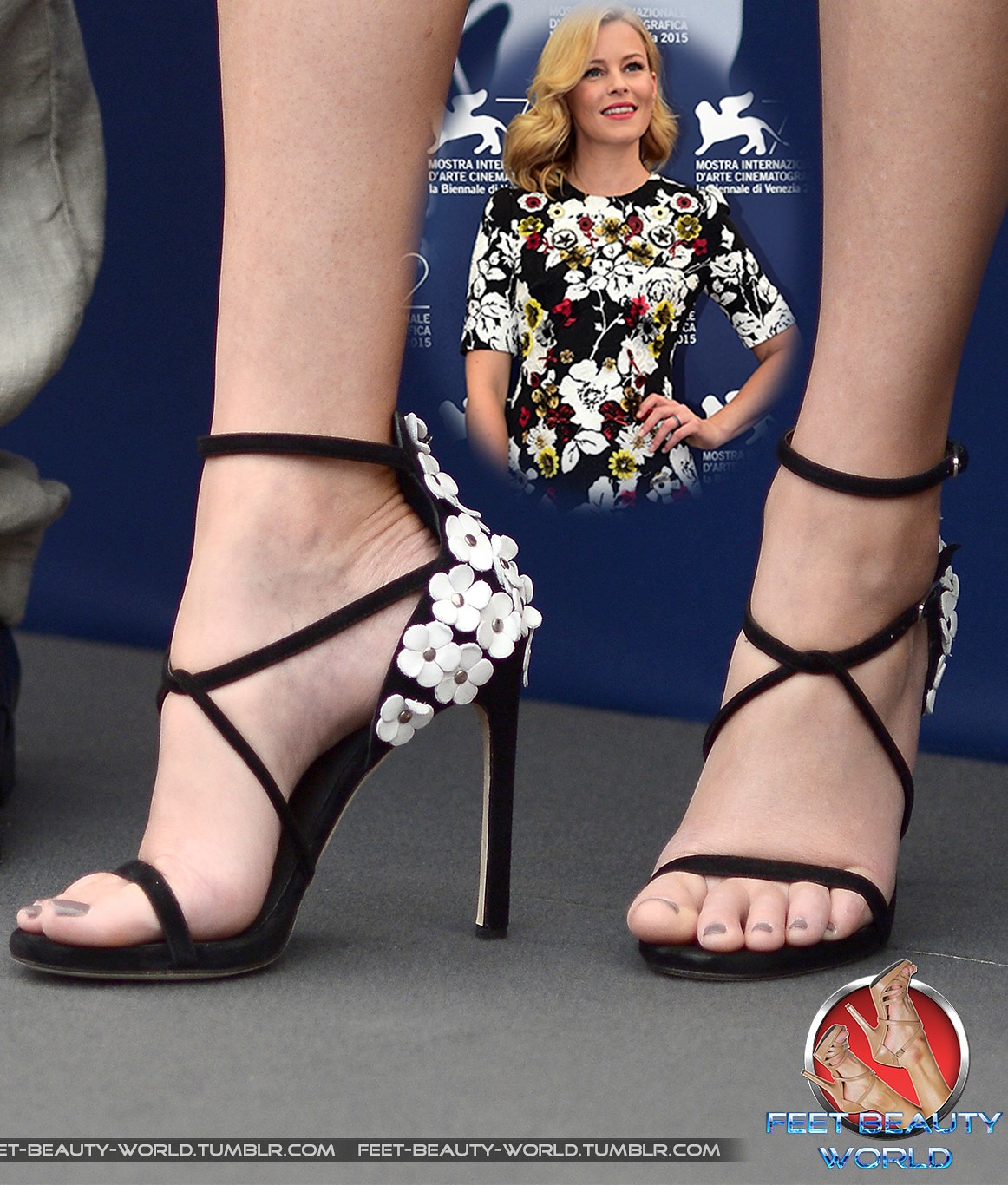The photograph is a carefully composed image featuring a close-up of a woman's feet adorned in black high heels, detailed with small white flower designs on the back. Her toes are painted with a grayish-brown nail polish, set against a gray carpet. Overlaid between her legs and feet is another photograph of the same woman, who is white with styled, wavy blonde hair, wearing makeup and a ring on her hand placed on her hip. She is dressed in a black dress with a vibrant floral pattern featuring colors like red, yellow, and white. The bottom left corner of the image features a watermark that reads "feet-beauty-world.tumblr.com," while the bottom right corner displays a logo within a silver ring alongside the same text, and showcases an additional pair of feet in beige heels. The detailed correlation between the woman's attire and her feet ties the image together, emphasizing her elegant presentation.